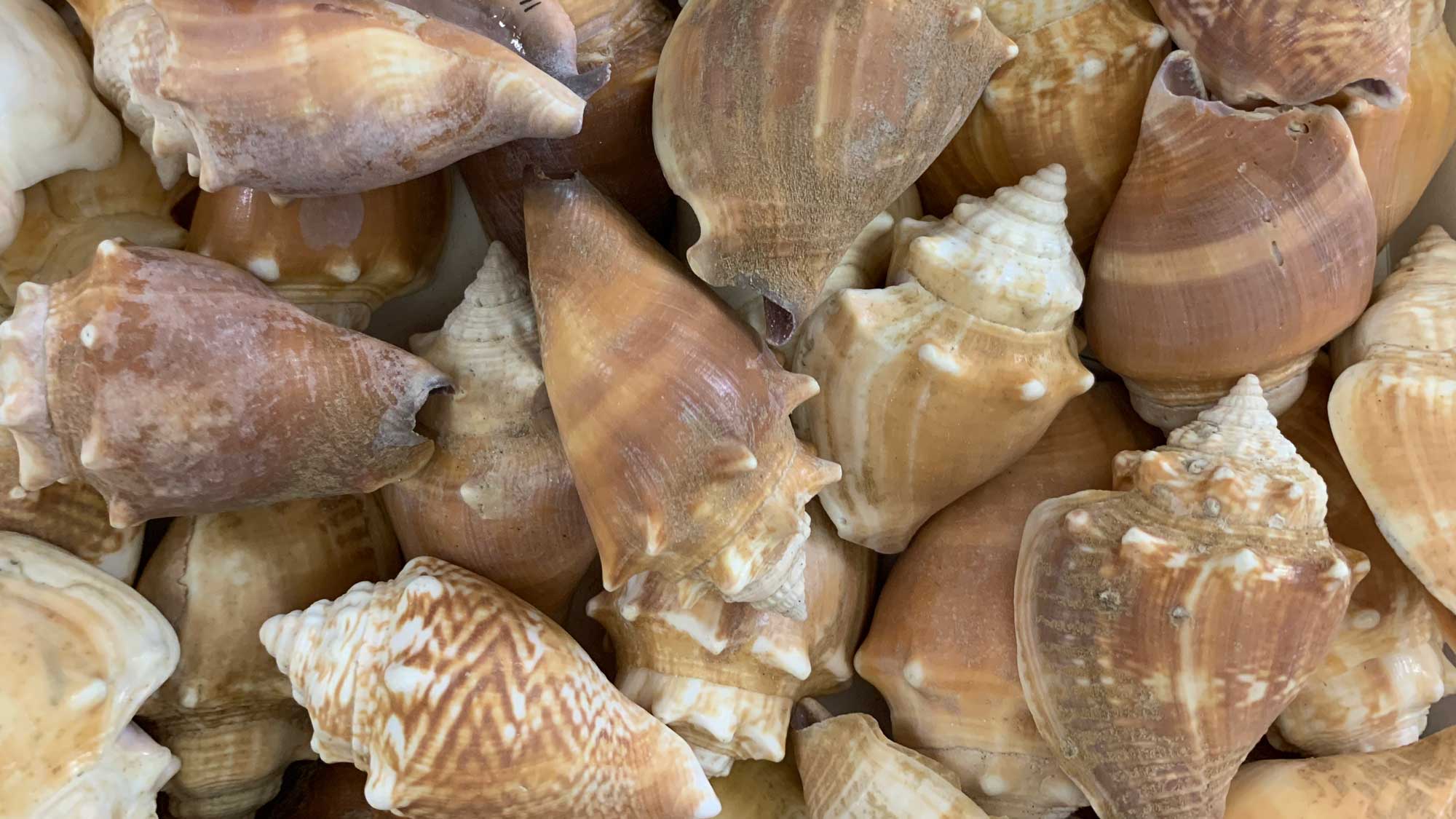This is a detailed color photograph showing an up-close view of a pile of over 20 conch shells, predominantly medium-sized, smaller than a hand but larger than tiny shells. The conch shells, characteristic of their traditional shape with a spiral of rings ascending to a sharp point at the top and curling around the bottom, exhibit a variety of natural wear indicative of time spent in the ocean. The shells display a harmonious palette of white, beige, brown, tan, and cream, with some featuring distinct patterns like stripes, wavy lines, and zigzags. Notably, the shell in the front center showcases a zigzag pattern blending white, tan, and brown hues, while the one at the bottom right stands out with its textured bumps and predominance of tan accented with white. The majority of the shells are empty, showing no visible creatures inside, and their surfaces display various conditions—from perfect to having tiny cracks—enhancing the intricate details of their ocean-worn exteriors.